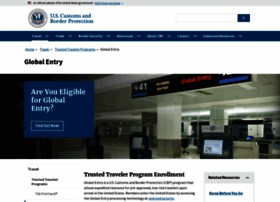A screenshot of a website featuring the US Customs and Border Protection main page. The image quality is low, rendering much of the text difficult to discern. At the top, a gray header spans across the page, followed by a white banner beneath it. Prominently displayed is a governmental emblem resembling a SEAL-style logo, flanked by the text "US Customs and Border Protection." To the right of this logo, there is a search bar with a blue search button.

Below this section lies a blue navigation bar featuring various options in white text accompanied by white dropdown arrows, but the small text size makes them illegible. The central part of the page showcases an image of people queuing, presumably at an airport, with a noticeable blue square box containing the text, "Skip the line with Global Entry."

Further down, there is an explanatory text section headed with, "Global Entry: Trusted Traveler Program Enrollment." However, the detailed body text is too small to read clearly. On the right-hand side of the page, there is a related content area with clickable links, although the specifics are also not clearly visible due to the image’s resolution.